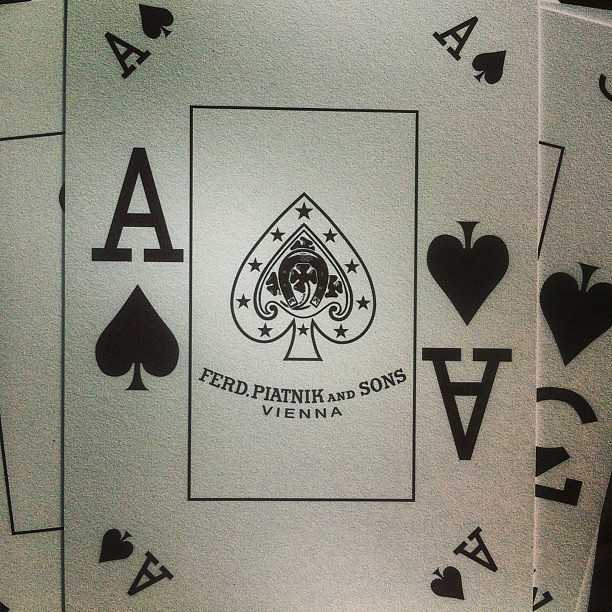The photograph features what appears to be a playing card or a design inspired by one. At first glance, it resembles a stack of playing cards, particularly highlighting an Ace of Spades card produced by Ferd Piatnik & Sons in Vienna. The design on the card exhibits a central spade symbol accompanied by an upside-down horseshoe. Below the spade, the text “Ferd. Piatnik & Sons” arcs gracefully, with "Vienna" inscribed underneath. Around the card's borders, traditional Ace of Spades markings include capital 'A's at the corners alongside smaller spade symbols. Notably, the surface texture appears grainy, though it is unclear whether this is due to the material of the card or the quality of the image itself. Surrounding the card are hints of fold lines and repeated patterns, suggesting it might be part of a larger object such as a handkerchief or tablecloth adorned with playing card designs. The colors on the white surface exhibit subtle grey, green, blue, and pink hues, further contributing to the enigmatic texture of the image.